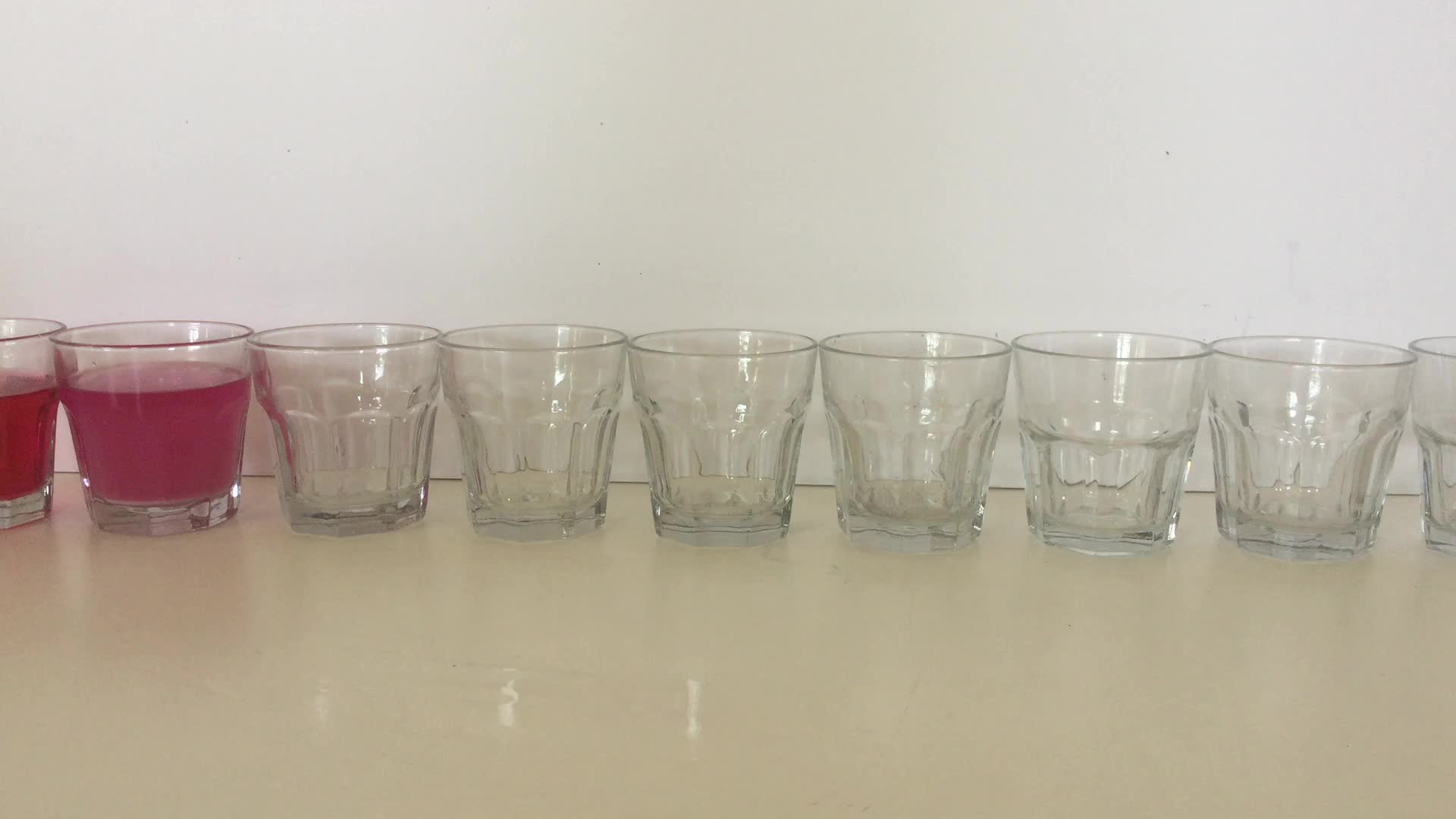This photograph depicts a row of ten small drinking glasses arranged horizontally on a smooth, tan-colored countertop at the base of a plain white wall. Each glass, flared at the top and narrowing towards the base, appears to hold about 8 to 12 ounces. The two glasses on the left contain a fruit punch or juice-like liquid, one showing a reddish color and the other a purplish hue, possibly altered by lighting. The remaining glasses, seven of which are fully visible while the last one is partially visible on the right edge of the frame, are empty and feature vertical ridges. Light reflections can be seen on the tan surface, particularly in the lower left corner of the image.